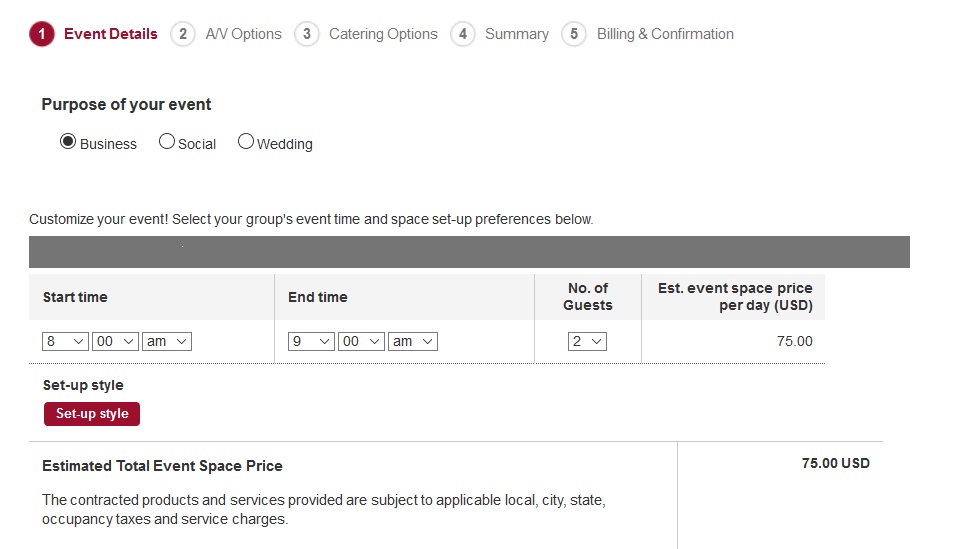The image depicts a detailed form being filled out to reserve an event space. The form itself is wide, indicating it is likely being viewed on a computer rather than a mobile device. The background is a plain white, giving the form a clean look.

The reservation process is divided into five distinct stages: Event Details, AV Options, Catering Options, Summary, Billing, and Confirmation. The particular stage currently displayed is "Event Details," highlighted in red, along with the number "1" inside a red circle, signifying it is the first step.

In this section, the purpose of the event must be indicated, with options including Business, Social, and Wedding. The individual has selected "Business." Below that, there are fields for customizing the event, such as selecting groups, event time, and space setup preferences.

The form specifies that the event will start at 8:00 AM and end at 9:00 AM, lasting for one hour. The expected number of guests is two, and the estimated event space price per day is noted as $75 USD. Below the timing details, there is a section labeled "Setup Style" within a red rectangle, although the particular style is not specified.

Further down, the form reiterates the "Estimated Total Event Space Price" at $75 USD, reminding users that the contracted products and services are subject to relevant local occupancy taxes and service charges.